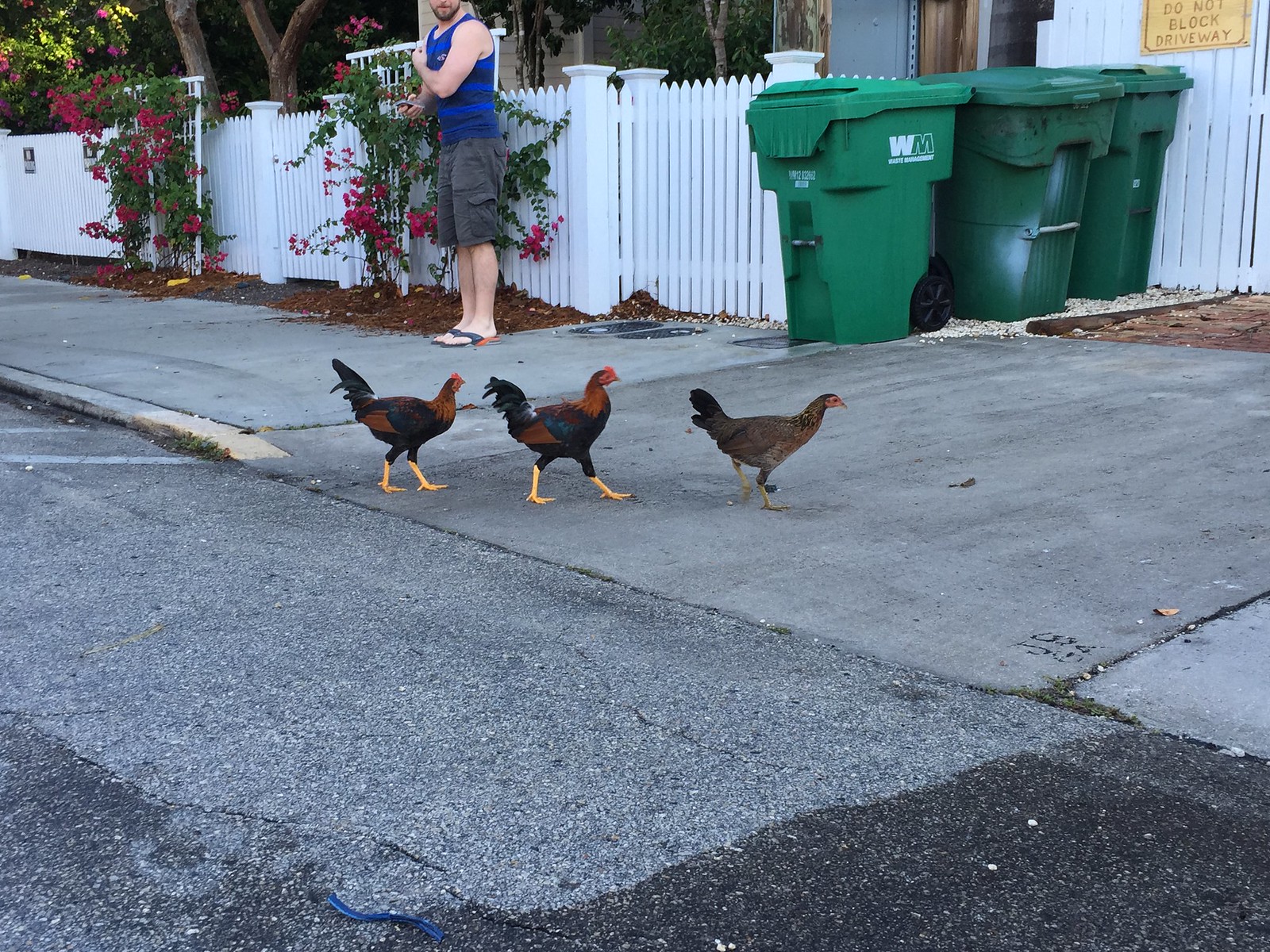In this outdoor scene, a fair-complexioned man wearing a blue tank top, gray cargo shorts, and flip-flops stands timidly by a white picket fence adorned with blooming rose bushes and vines on a trellis. His left hand crosses his body as he observes three chickens walking single file across a sidewalk that converges with a driveway partially made of brick and asphalt. The chickens include one light brown, one black and red, and one primarily brown and red. In the background, trees and houses are visible, as well as a curb and street to the left of the sidewalk. Three green plastic trash cans are lined up near the white fence, which also bears a "Do Not Block Driveway" sign. The man's face is not fully visible, showing only his chin, which conveys a somewhat scared expression. The chickens, featuring notable details such as yellow legs and red caps on two, appear content as they move across the driveway.